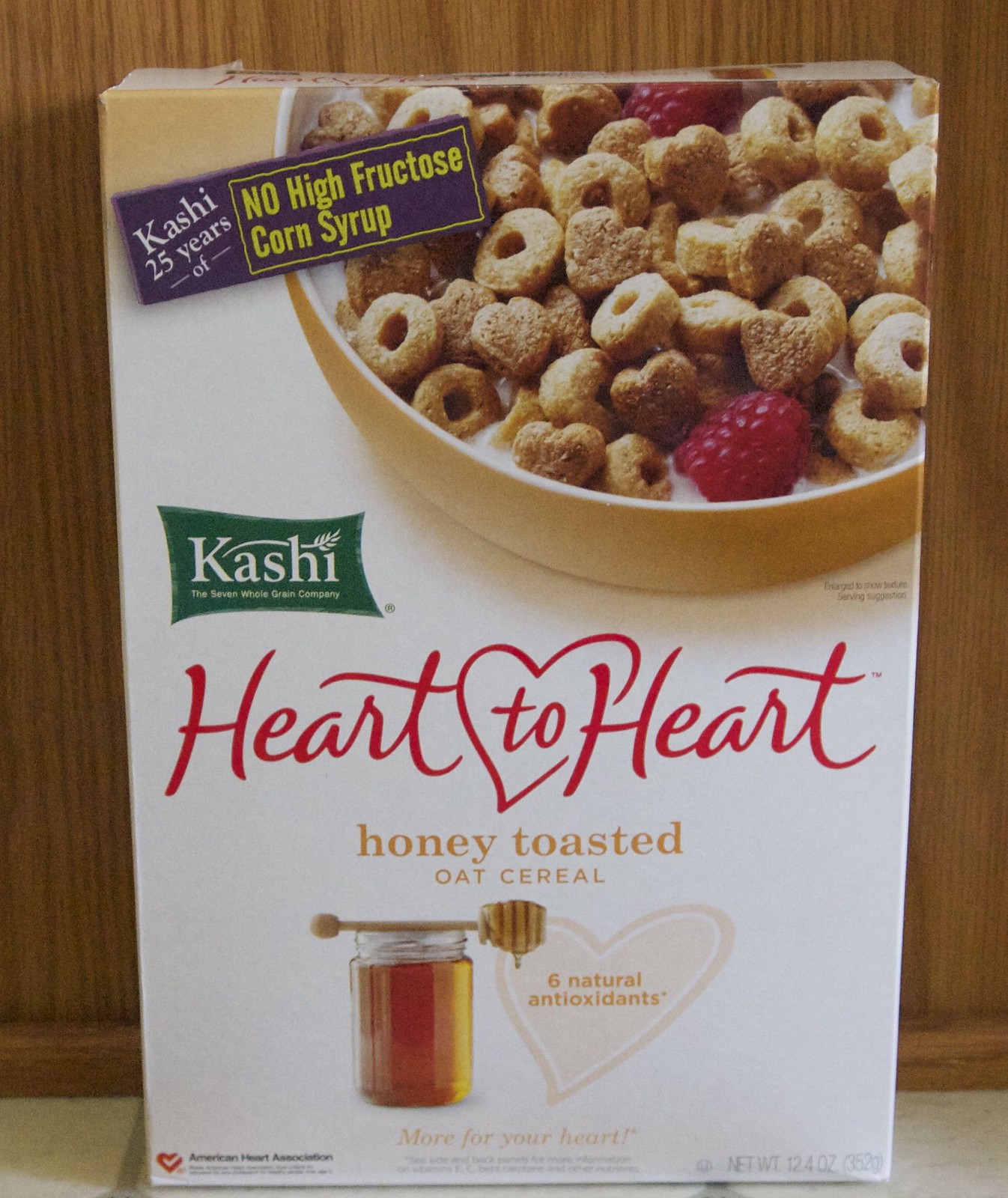The image depicts a vertically aligned, rectangular photograph of a cereal box placed on what appears to be a white tile surface, with gray grout visible between the tiles. The background features a brown cabinet with visible wood grain lines. The cereal box, which occupies the majority of the frame, is branded by Kashi, identifiable by a green, curved rectangular logo located towards the left center of the box. The logo features white text and a small grain illustration. Below the logo, the name of the cereal, "Heart to Heart," is written in large, red letters, with "Honey Toasted Oat Cereal" in gold text beneath it. 

The top portion of the cereal box showcases a large image of a yellow bowl filled with the cereal, which includes circular whole-grain pieces similar to Cheerios and some heart-shaped pieces, with several raspberries mixed in. Adjacent to this image, a blue and yellow rectangular section highlights "Kashi, 25 years of no high fructose corn syrup." Additional details include a small honey jar with a honey wand depicted towards the bottom center, along with a heart symbol containing the text "six natural antioxidants." The bottom of the box provides further information about the cereal's weight and association with the American Heart Association.